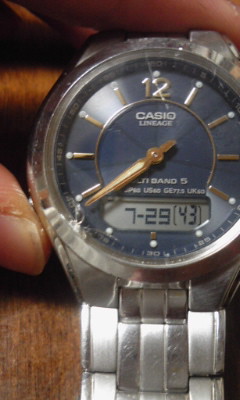The image depicts a close-up view of a Casio Lineage wristwatch, held delicately between someone's thumb and index finger. The watch face is a deep, dark blue, highlighted with gold elements. The only numeral visible on the face is the number '12' in gold at the top, while the remaining hour indicators are represented by elegant gold lines with white dots. The hour and minute hands are also gold, with the hour hand notably shorter than the minute hand. Across the face, there are visible imperfections: scratches angle through the '12' and there's a crack at the bottom left of the face. The sunburst design, formed by the gold outline at the center with radiating lines, adds a striking visual effect. Below, a small rectangular digital screen displays the date as '7-29' and '43' seconds. The time on the analog portion matches the digital readout at 7:29. The watch band and casing are made of silver chain links, adding a classic contrast to the dark blue face. Overall, the image combines the elegance of the watch with the reality of its wear, captured in a moment of detailed examination.